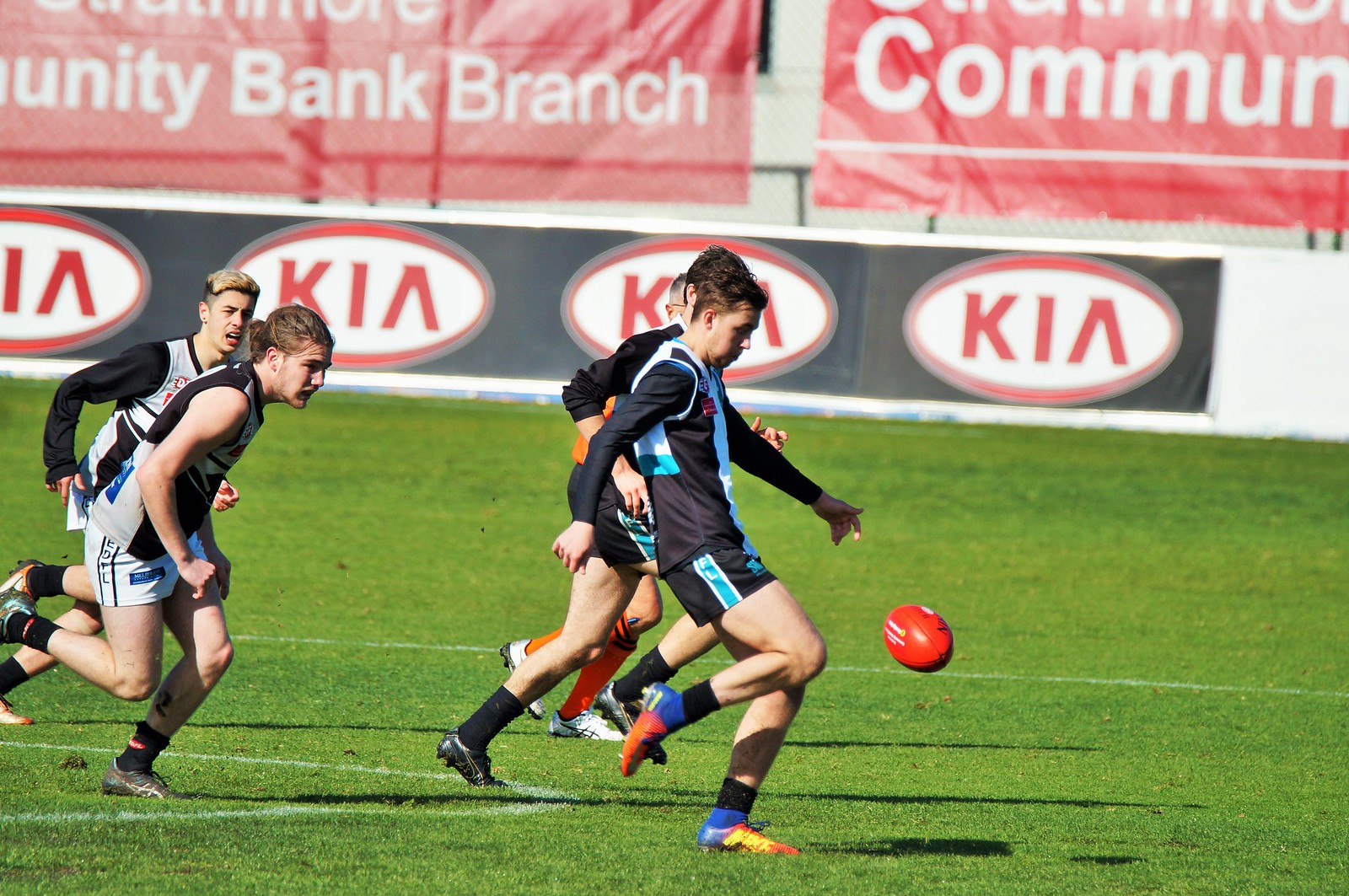The image depicts four young men, likely in their early twenties and all appearing to be white, engaged in what seems to be either a rugby or soccer match on a green field under clear daytime skies, with the sun shining brightly on them. The players are heading to the right, and one player in the foreground, who has orange and blue cleats, is poised to kick a ball that appears to be either a rugby or a red soccer ball. Two of the players have distinctive hair; one has bleached hair and another has his hair pulled back into a ponytail or bun. The players are in varied uniforms, some in black shorts with a blue stripe and matching black tops, and others in white shorts. One player is notably wearing a sleeveless shirt. The background features a series of repeating banners: a black one showcasing the red and white Kia logo, and a red one with partially visible white text, reading "Community Bank Branch."